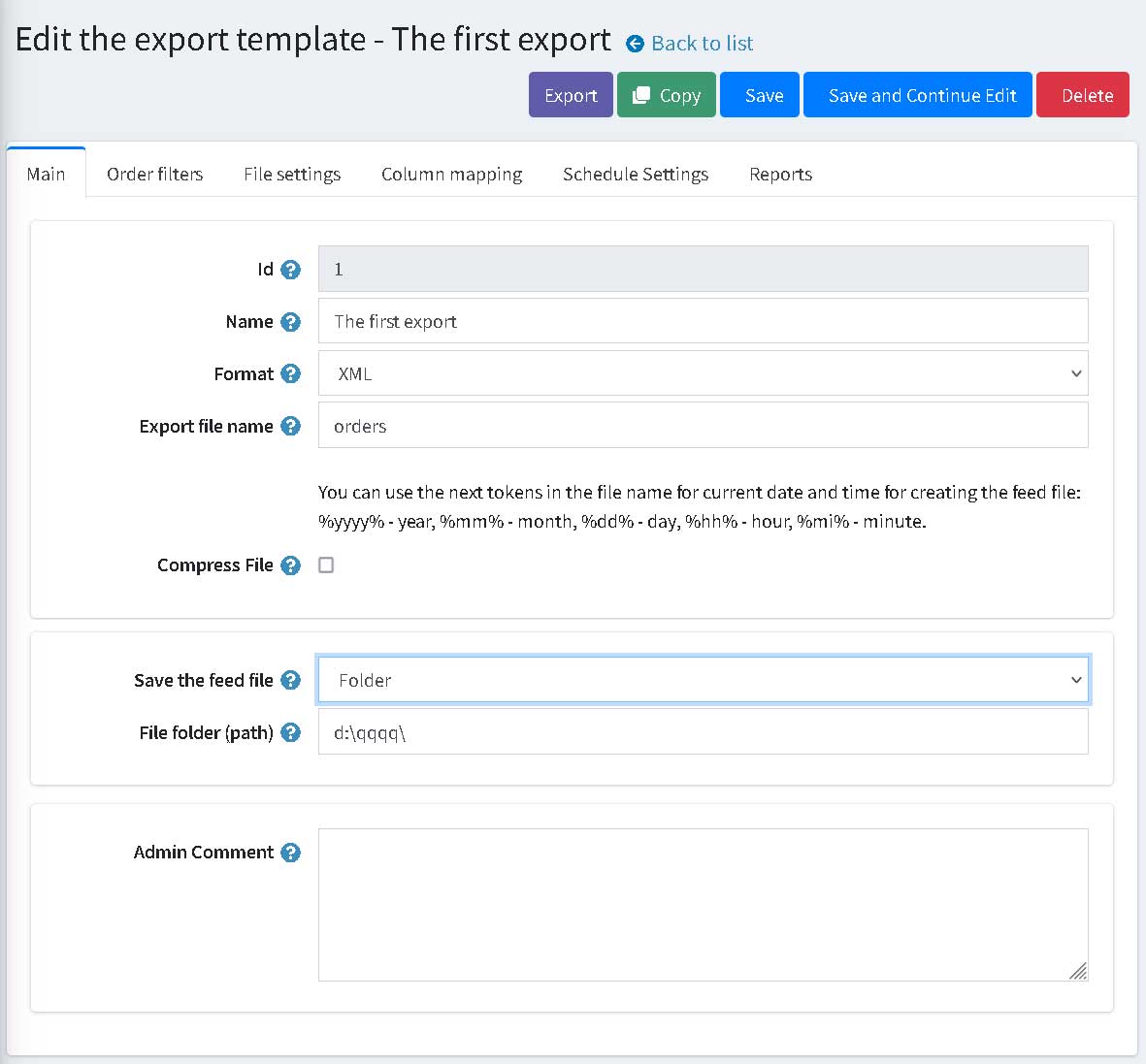This image is a screenshot of a form interface used for editing an export template. 

In the upper left corner, a gray background spans from the upper left to the upper right with the heading "Edit the Export Template." Adjacent to the heading is a blue back arrow labeled "Back to List," which is a clickable live link. Below this header are several buttons arranged horizontally: a purple "Export" button, a green "Copy" button, a blue "Save" button, a blue "Save and Continue" button, a red "Edit" button, and a red "Delete" button.

Beneath this section, the form interface itself is displayed with a white background. There are multiple tabs at the top: "Main," "Order Filters," "File Settings," "Column Mapping," "Schedule Settings," and "Reports." The "Main" tab is currently active, indicated by a blue line above it.

In the "Main" tab, there is a form to be filled out with several fields. The "ID" field has a gray background with the number "1" entered. The "Name" field has "The First Export" typed in. The "Format" field contains "XML." The "Export File Name" field shows "orders." A note beneath this field states that certain tokens can be used in the file name to include the current date and time for creating the feed file. Various codes are listed presumably for this purpose.

Below these fields, there is an option labeled "Compress File" which is not checked off. Another option, "Save the Feed File," is highlighted and centered in blue. The user has selected a folder for this, indicated by a down arrow beside a file icon. Finally, the "File Folder Path" field contains the path "D:\\QQQQ\\." There is also an "Admin Comment" section visible but not filled out.

This detailed description encapsulates the structure and content of the form as shown in the screenshot.